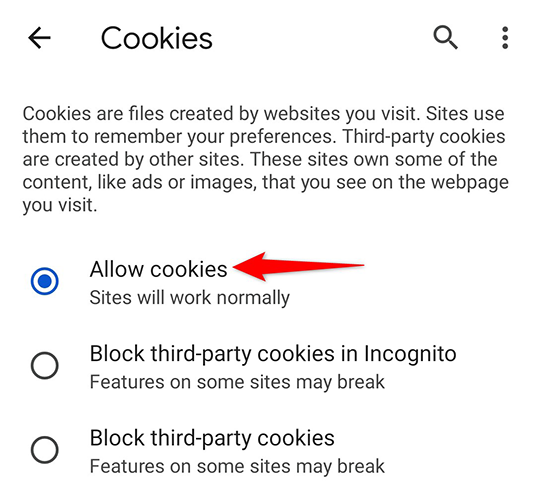**Image Description: A Guide to Cookie Settings**

The image features a white background with black text and various graphical elements designed to explain the concept of cookies and user preferences for managing them.

- **Top Section:**
  - **Left Arrow Icon:** Positioned at the top-left corner, pointing towards the left, with the text “Cookies” next to it.
  - **Magnifying Glass Icon and Three Dots:** Located nearby, indicating additional options and search functionality.

- **Main Text:**
  - **Title:** "Cookies" - A brief introduction explaining that cookies are files created by websites you visit for remembering your preferences.
  - **Description:** "Cookies are files created by websites you visit. Sites use them to remember your preferences. Third-party cookies are created by other sites. These sites own some of the content, like ads or images, that you see on the web page you visit."

- **Options for Cookie Management:**
  - **Allow Cookies:** Represented by two nested blue circles, with the text “Allow cookies” written inside. A large red arrow points to this option along with the note: "Sites will work normally."
  
  - **Block Third-Party Cookies in Incognito:** Represented by a black circle with a white fill, containing the text “Block third-party cookies in incognito.” A note below mentions: "Features on some sites may break."
  
  - **Block Third-Party Cookies:** Another option symbolized by a black circle with a white fill, with the text “Block third-party cookies.” Similar to the previous option, this one also includes the note: "Features on some sites may break."
  
- **Summary:** Users have the choice to allow cookies, block third-party cookies in incognito mode, or block third-party cookies altogether. These settings influence how sites track your activity and how some site features may function.